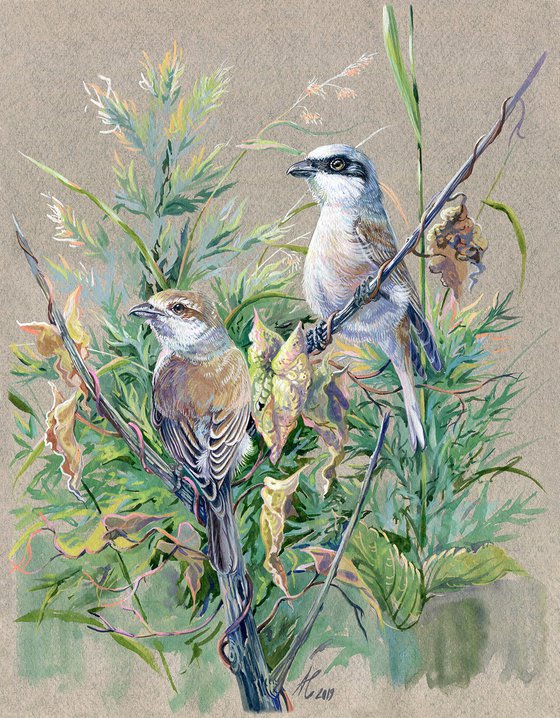The photograph captures a rectangular painting featuring a detailed natural scene. The background, a canvas-like material in varying shades of light grayish-brown and gray-blue, sets a serene tone. Central to this painting are two distinct birds perched on intertwining branches adorned with lush foliage in various shades of green. The bird on the left showcases a mix of black tail feathers, brown-spotted wings tipped with white, a white neck, and a brown head, completed by a light gray curved beak. In contrast, the bird on the right is predominantly white on its front and head, with a striking black stripe across its eyes resembling a blindfold, ending with a curved black beak and dark brown wings and tail feathers. Both birds gaze towards the left of the painting. The branches they sit on are not solitary but part of a larger growth with light green leaves and some possibly flowering elements displaying yellow or peach hues. Towards the top of the painting, there are white and green leafy elements. Below, a small, unreadable signature marks the artist's identity. The entire setup exudes a watercolor-like soft and naturalistic charm, making the birds and the flora look vibrantly lifelike.